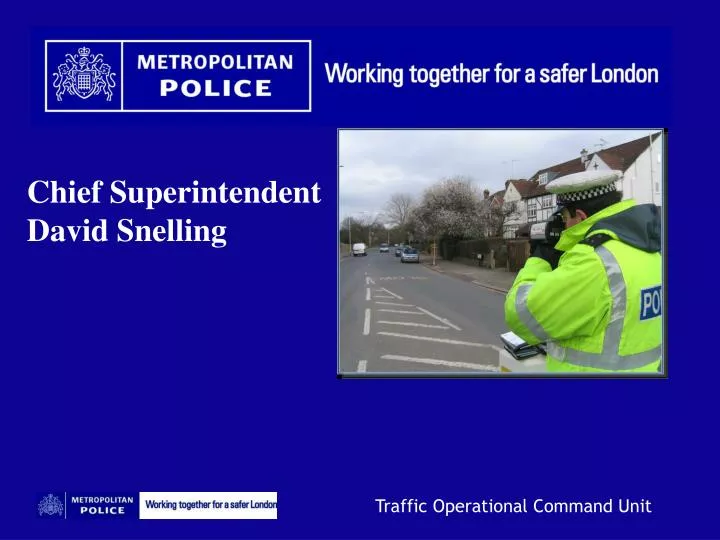The image features a solid blue background with prominent white text. At the top left, the Metropolitan Police logo is displayed along with their tagline, *Working Together for a Safer London*. Below this, on the middle left, the text reads *Chief Superintendent David Snelling*. The focal point on the right side of the image is a photograph of a police officer standing on a street. The officer, wearing a yellow police vest and a white hat, is aiming a speed radar gun at traffic under an overcast sky. The scene features several parked cars on the sidewalk and a white building in the background. Trees and fences line the road. At the bottom left of the image, the caption reads *Metropolitan Police* alongside the tagline *Working Together for a Safer London* and the designation *Traffic Operational Command Unit*.